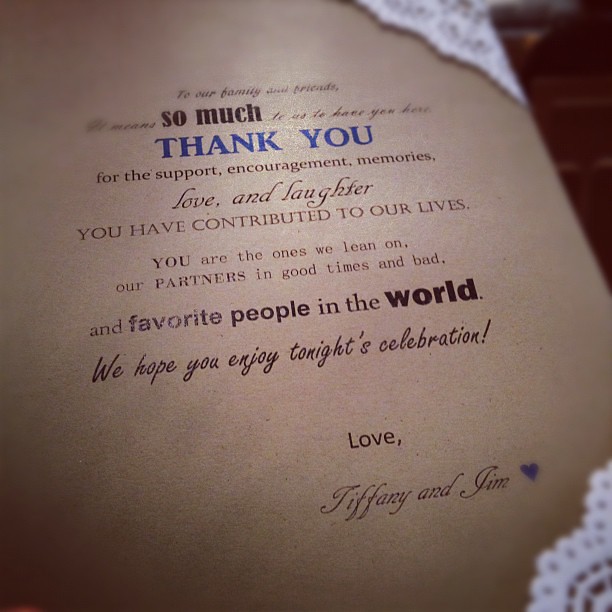This square, 5-inch by 5-inch photograph features a thank you note the size of a place card, printed on brown cardstock, and positioned on a similarly colored table. The note is at a slight leftward tilt, clearly showing the upper right-hand corner. Small white doilies embellish both the upper and lower right-hand corners of the cardstock, adding a touch of elegance. The message on the card begins at the top center in small black cursive with "To our family and friends." Following this, the phrase “so much” stands out in bold black print. It continues in cursive with “to us to have you here.” A prominent bold blue "Thank you" catches the eye next. Subsequent text in smaller black print reads: "For the support, encouragement, memories, love, and laughter you have contributed to our lives. You are the ones we lean on, our partners in good times and bad, and favorite people in the world." In cursive, the note concludes with, "We hope you enjoy tonight's celebration. Love, Tiffany and Jim," accompanied by a small purple-blue heart. The combination of varied fonts and colors, along with the intricate doily decorations, suggests that this thank you note is likely part of a special celebration, possibly a wedding.